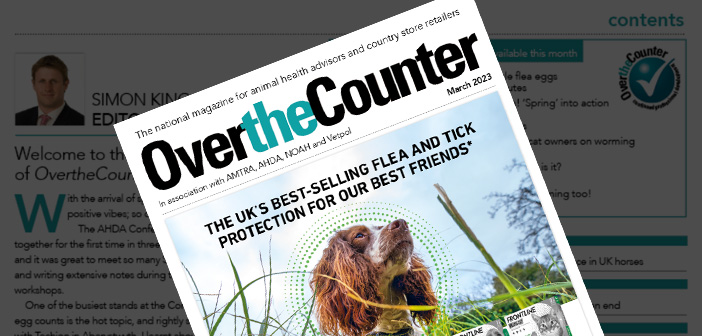This image showcases a computer screen displaying a digitally overlaid magazine cover atop another page. The background features a grayscale image of a man with text next to him that reads "Simon, K-I-N" along with an illegible article title. In the upper right corner, the word "contents" appears in light green amidst the gray haze. 

The prominent magazine cover in the foreground is titled in small black letters, "The National Magazine for Animal Health Advisors and Country Store Retailers." Boldly displayed, the title reads "Over the Counter," with "the" highlighted in teal. Additionally, the cover notes its affiliation with organizations such as AMTRA, A-H-D-A-N-O-A-H, and V-E-T-P-O-L, dated March 2023. 

The central image on the magazine cover features a close-up of a spaniel's head, characterized by reddish ears, red facial markings, and white fur. Surrounding the dog's head are green dots and a backdrop of grass, alongside the caption, "The UK's best-selling flea and tick protection for our best friends."